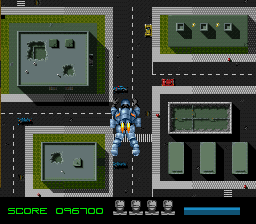This image appears to be a still from a video game, presenting a character adorned in a bulky suit of chrome and silver-colored body armor, complete with a helmet that obscures any visible skin. Positioned centrally, but slightly lower in the image, the character is depicted in a skydiving pose, mid-jump, with a jetpack on their back emitting vibrant yellow and orange flames. Below the character is an aerial view of a simplistic, digitally rendered town featuring four large buildings on distinct blocks, equipped with utilities like air conditioning units and a trio of chimneys on one. The black streets below, marked with white dashed lines, are traversed by yellow, red, and blue vehicles. A black band runs across the bottom of the image, displaying green text that reads "score 096700." Alongside this score, there are four icons representing the protagonist's remaining lives and a blue status bar. The overall visual style is angular and distinctly digital, emphasizing a non-hyper-realistic aesthetic.